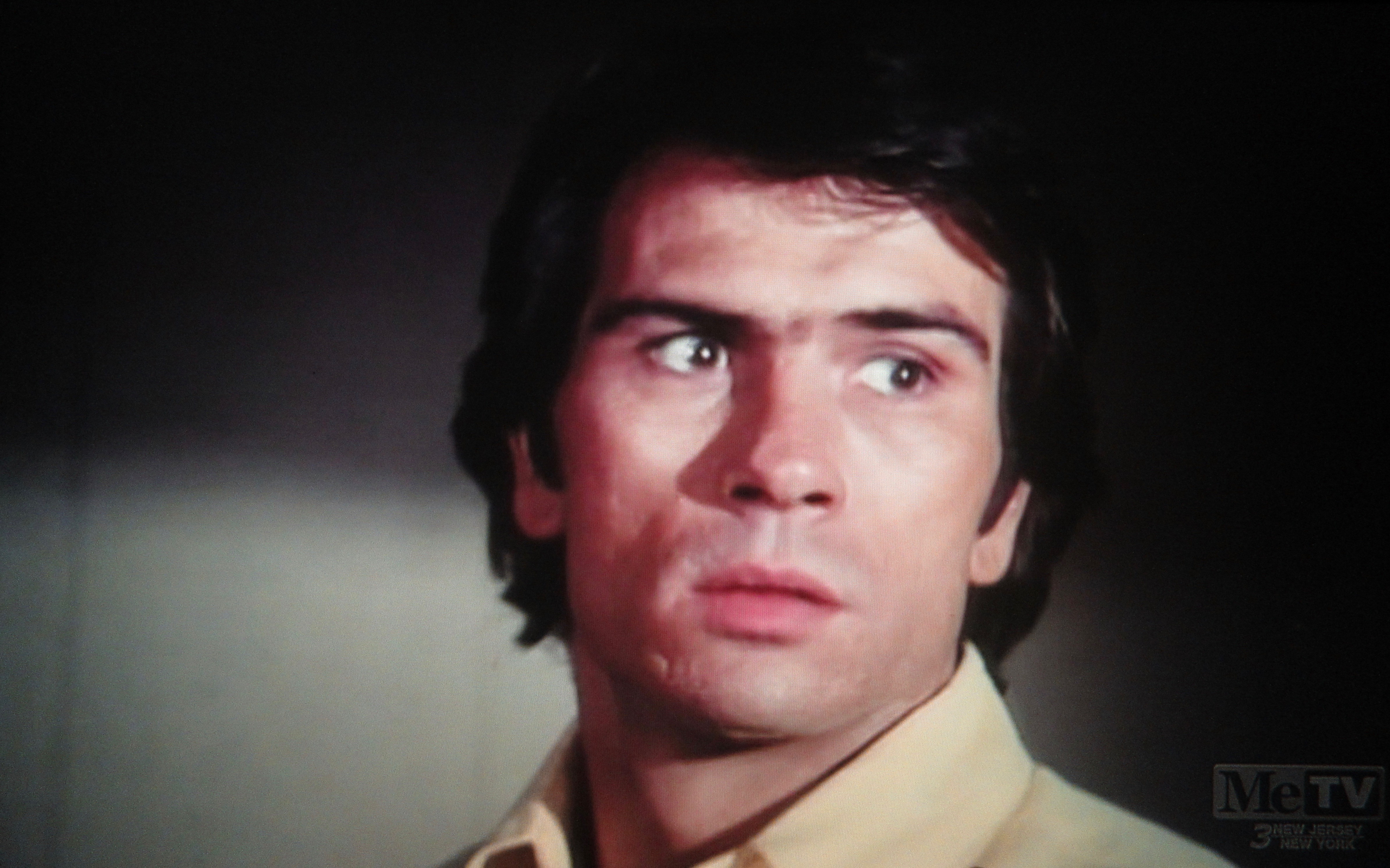The image is a color photograph in landscape orientation, prominently featuring a close-up of a man in his 30s or early 40s. He has a slightly square chin and dark, fluffy brown hair, styled in an 80s look that reaches down to his neck. The man is wearing a light yellow or cream-colored button-up shirt with the top button undone. His nervous expression is directed towards the bottom right corner of the image, where his eyes seem fixated on something off-screen. The background consists of a white wall, which appears lighter on the left side and darker on the right, intertwined with multiple creases or lines. The quality of the image is somewhat low resolution, adding a grainy texture to the photograph. Additionally, a semi-transparent watermark that reads "MeTV, 3, New Jersey, New York" is situated in the bottom right corner. There is also an out-of-focus light shelf or cabinet with vertical panels in the bottom left corner, contributing to the overall scene of the photograph.